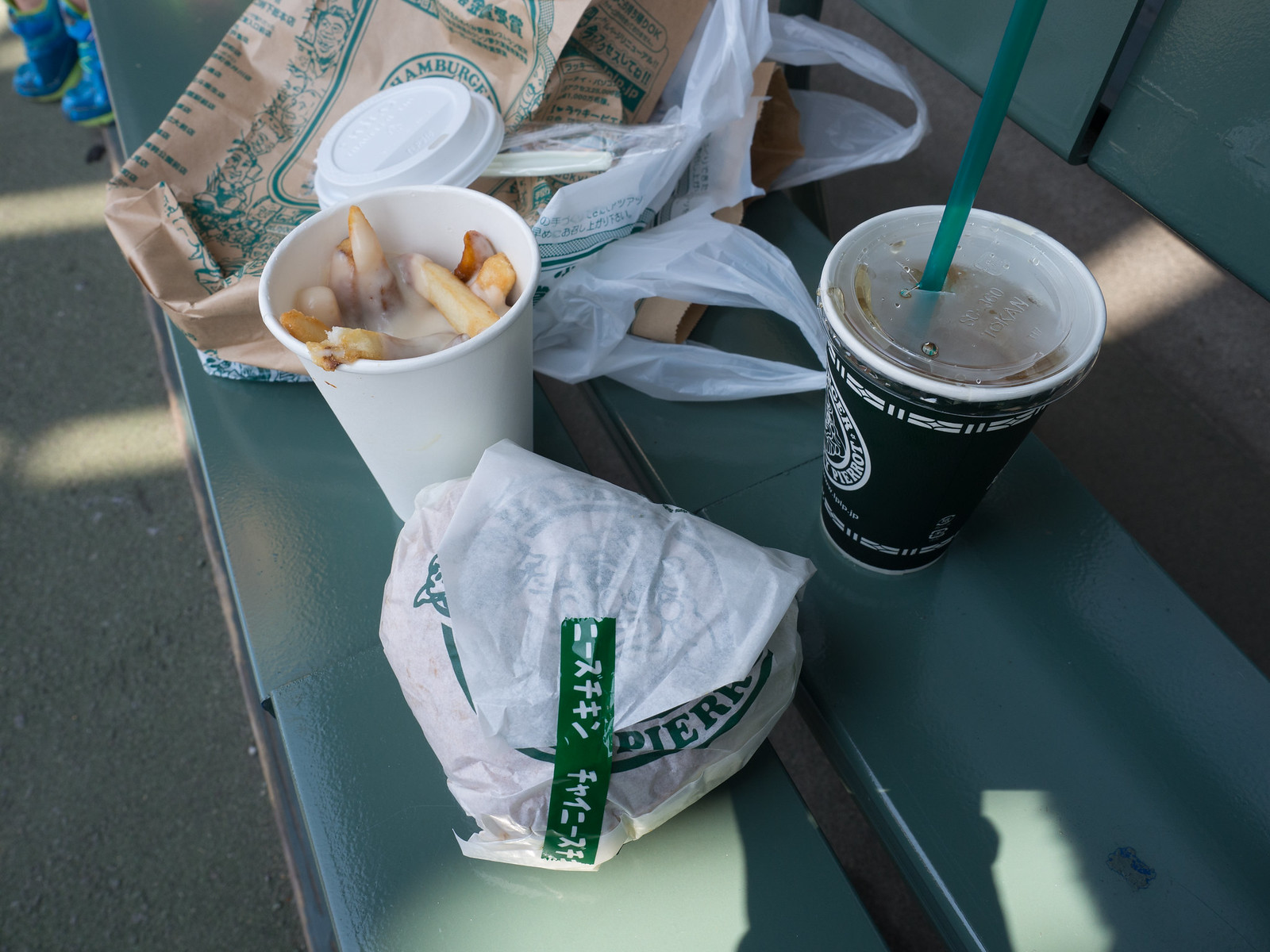The image showcases a close-up of a dark green park bench covered with various fast-food items. Centered on the bench is a wrapped sandwich sealed with a green sticker. Beside it is a cup filled with fries topped with a white creamy substance, potentially a sauce, all contained in a white cup. To the right, there is a black cup of soda with a clear plastic lid and a green straw sticking out, featuring the text "P-R-E-R-R-O-T". In the background, there's a brown paper bag adorned with the restaurant's branding and a white plastic bag. A coffee lid and a plastic spoon rest casually amongst the items. The ground beneath the bench is a coarse, dark gray gravel, with a hint of blue boots visible at the top left corner. The setting appears to be outdoors, perhaps in an area close to a fast-food restaurant.